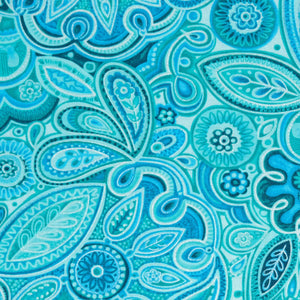This square image showcases an intricately illustrated psychedelic paisley pattern dominated by teal, light blue, and white hues. The ornate design features a variety of shapes, including stylized flowers, leaves, teardrops, and ovals, all intricately detailed with internal patterns and enhanced by different shades of blue. Prominently, in the bottom left corner, there's a dark blue and light blue leaf shape filled with white line drawings of smaller leaves. Nearby, a stylized sunflower with dark blue petals and a white center is encircled by white lines. Towards the right, a light blue feather with interior blue and light blue leaves can be found. The upper left corner houses a large flower with accompanying leaves and petals. Tightly packed with decorative elements, the background peeks through in spots, mostly in white, accentuating the overall teal and light blue color scheme. The composition suggests a potential textile or fabric design, rich in psychedelic and paisley motifs.